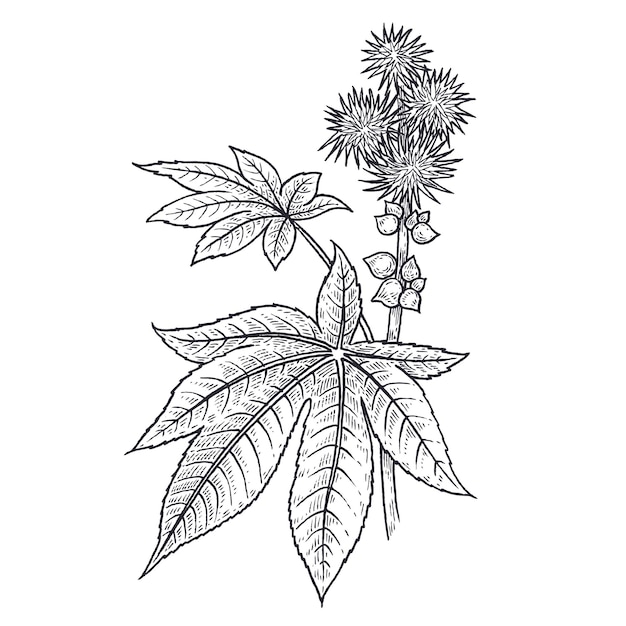The image is a black and white sketched drawing of various leaves and flowers set against a solid white background, without any text or borders. In the top right corner, there are four spiky, bulb-like flowers attached to a stem that extends diagonally downwards to the bottom right. Surrounding these flowers are small, teardrop-shaped leaves. Towards the center of the image, small petals are clustered together. On the left side, there is a large leaf with a stem that extends to the middle of the image. This leaf has a distinct, elongated oval shape with pointed tips and curved horizontal lines running across it. In the lower half of the image, a very large, multi-sided leaf with six prominent sides takes up most of the space. There are also seven smaller leaves attached to the same branch, each oval-shaped with pointed ends. The overall style is consistent with a detailed botanical illustration, designed to be potentially colorable.